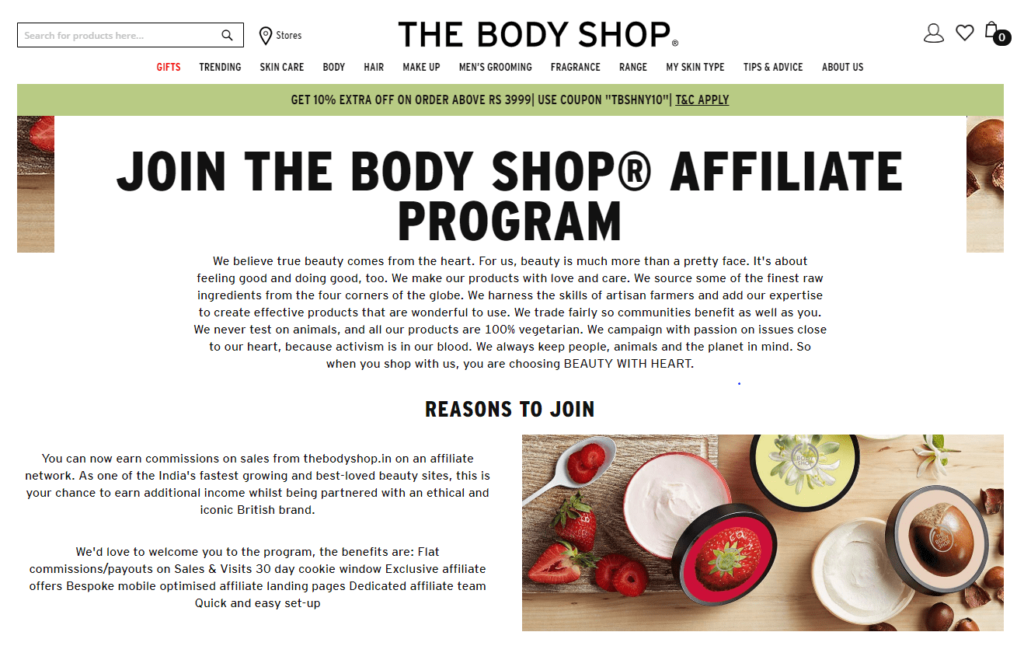The screenshot captures a promotional page from The Body Shop’s official website. At the very top, the header features a clean white background with 'THE BODY SHOP' written in bold, black, capital letters at the center. Below the header, there is a horizontal navigation menu. From left to right, the menu items are: 'Gifts' in red font, followed by 'Trending', 'Skin Care', 'Body', 'Hair', 'Makeup', 'Men's Grooming', 'Fragrance', 'Range', 'My Skin Type', 'Tips and Advice', and 'About Us', all in standard black font.

Underneath the menu, a pale green banner displays a special offer: "Get 10% extra off on orders above RS-3999, use coupon TBSNY10." To the right of this message, the text "T&C apply” indicates that terms and conditions are applicable.

Further down, on a white background, a large headline in bold, black, capital letters reads: "JOIN THE BODY SHOP AFFILIATE PROGRAM." Directly below, there's a brief description outlining the program, followed by a smaller headline, "REASONS TO JOIN."

On the lower right-hand side of the image, there is a top-down photograph showcasing an assortment of The Body Shop products, alongside fresh strawberries, suggesting that one of the products could feature a strawberry fragrance or ingredient. On the left side of the image, additional text explains the affiliate program in more detail, highlighting that participants can earn commissions on sales generated through The Body Shop's affiliate network.